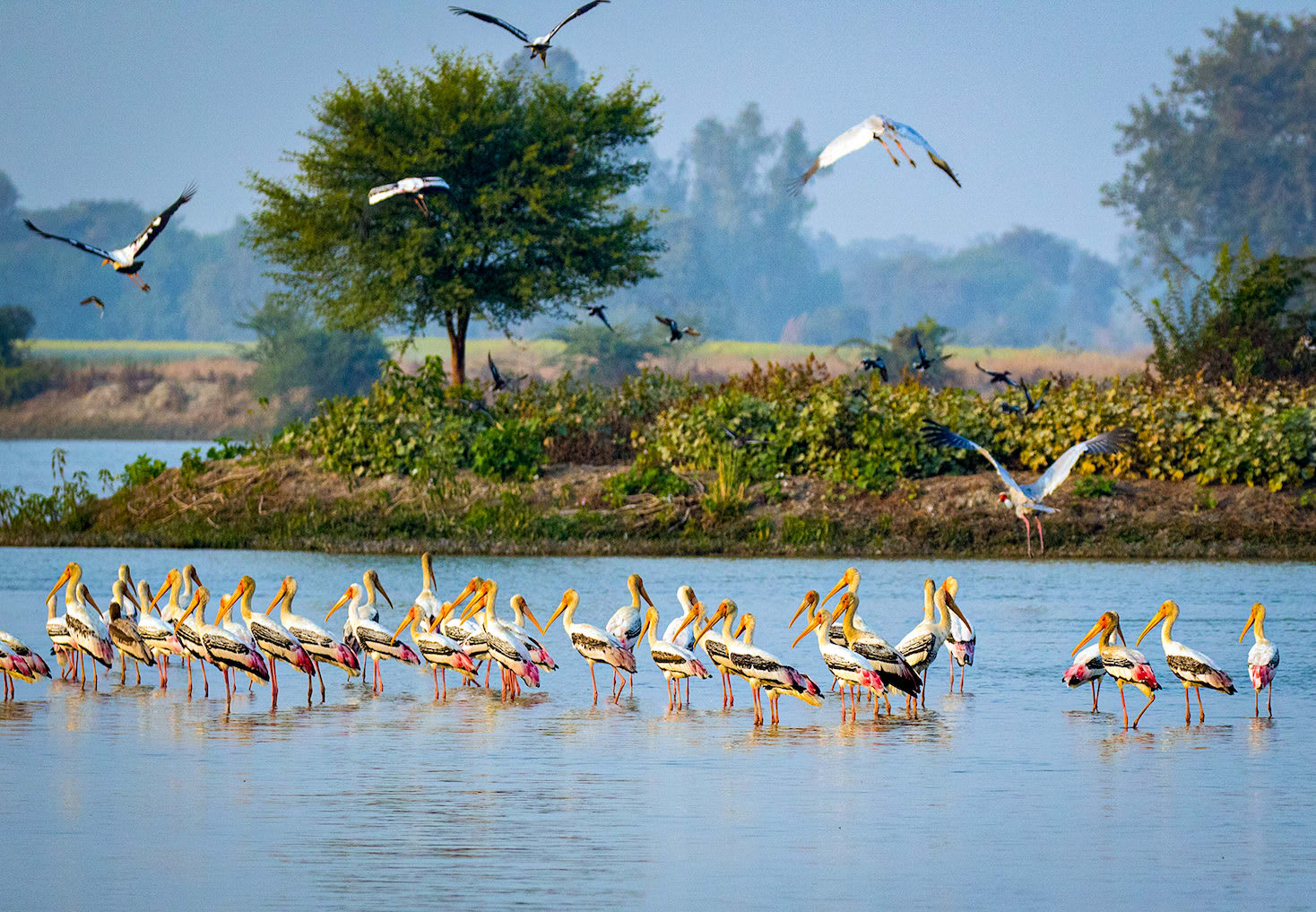The vibrant wildlife photograph captures a serene lakeside scene in what appears to be a lush, tropical environment. The foreground is dominated by a tranquil lake, on the surface of which stands a striking flock of approximately 20-30 storks. These storks, adorned with colorful plumage, display white backs, black wings, and bright pink tails, accompanied by distinctive orangish-yellow heads and beaks, and yellowish legs. The lively scene features the storks both wading in the shallow water up to their legs and taking to the sky in various stages of flight—landing, taking off, and soaring towards nearby treetops. 

Beyond the lake stretches a verdant landscape with low vegetation, shrubs, and a medium-sized, spreading tree, resembling a crepe myrtle, against a backdrop of richly forested hills and a clear blue sky. The distant shorelines and hills create a sense of depth, despite the slight blur, further emphasizing the dynamic presence of the storks in the immediate foreground. The overall scene exudes a sense of natural beauty and tranquility, highlighted by the storks' captivating colors and actions.